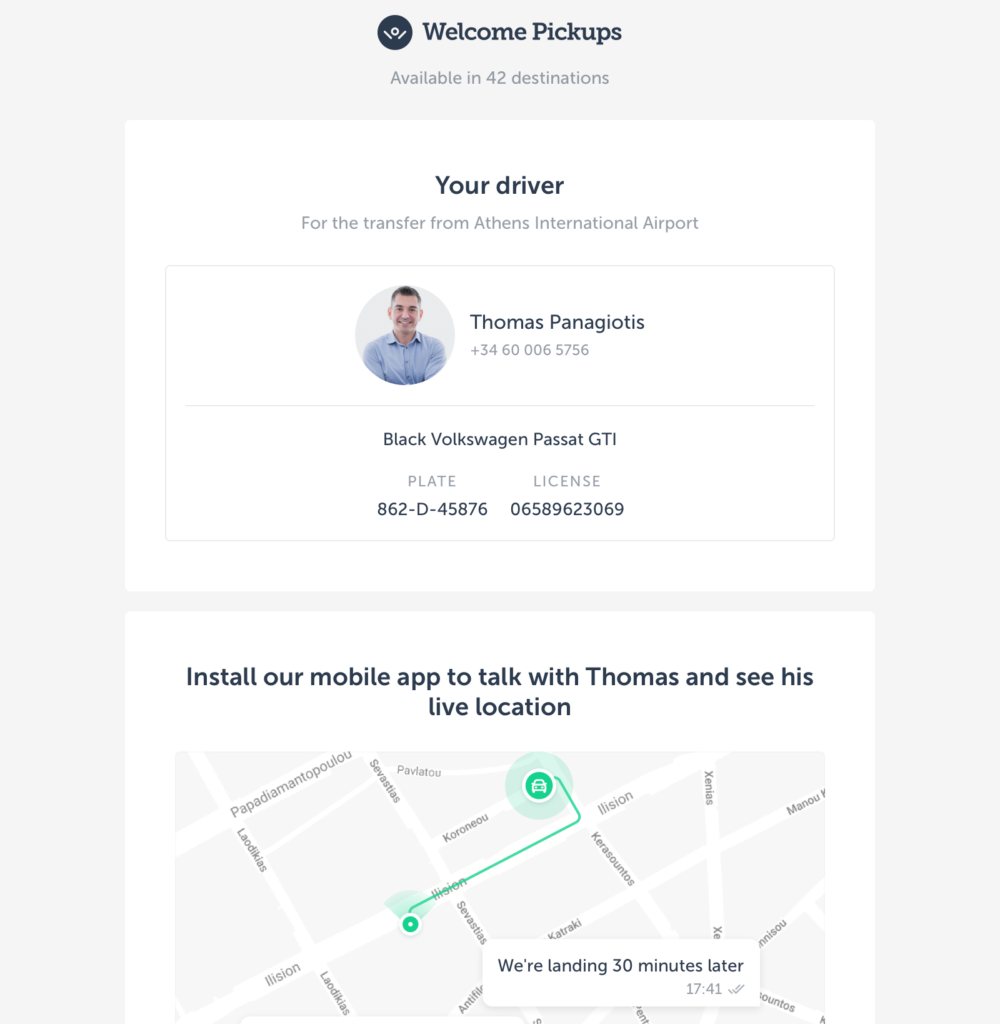Upon arrival at Athens International Airport, you will be greeted by your designated driver, Thomas Panagiotis. He will be driving a Black Volkswagen Passat GTI, with the license plate number 862D-45876 and personal license number 06589623069. His contact number is +3460-006-5756. Thomas is part of our "Welcome Pickups" service, which is available in 42 destinations. You can install our mobile app to communicate directly with Thomas and track his live location. Some of the destinations covered by this service include Ellison, Laudikus, Sevastias, Xenias, Claudia Green, White, and Black. Please note that our flight is scheduled to land 30 minutes later than originally planned.